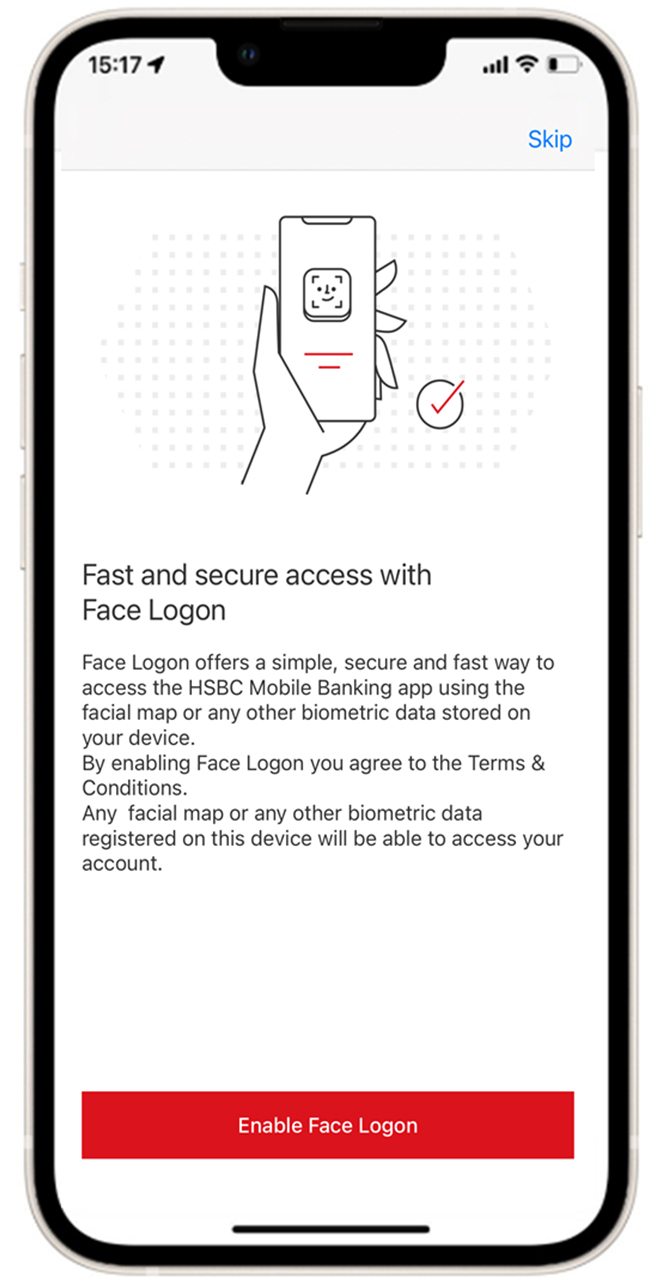The image prominently features a smartphone, depicted at nearly actual size. On the top left corner, the time is displayed as 15:17. Adjacent indicators show Wi-Fi strength, signal strength, and battery life. On the top right, there is blue text reading "Skip." Below this, an illustration of a person holding a smartphone with a smiley face in the center is visible. To the right of this illustration is a circle containing a red tick mark.

Directly beneath this, large text reads, "Fast and secure access with Face Login." Further down, smaller text provides more details about the feature: "Face Login offers a simple, secure, and fast way to access the HSBC Mobile Banking app using the facial map or any other biometric data stored on your device. By enabling Face Login, you agree to the terms and conditions. Any facial map or any other biometric data registered on this device will be able to access your account."

Towards the bottom of the image, still within the bounds of the smartphone, a large red rectangular button bears the white text "Enable Face Login."